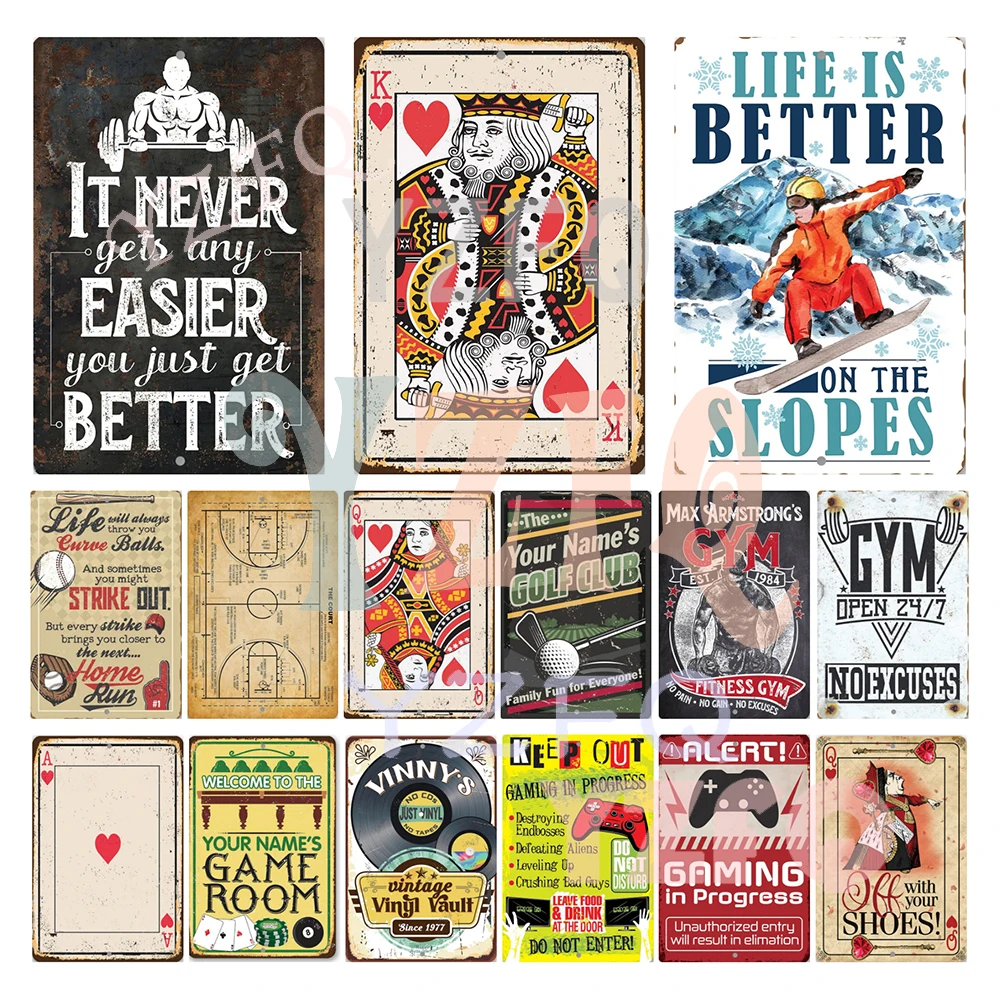The image is a collage of vintage-style, worn tin signs and posters that you'd typically find in someone's garage or game room. On the top left, there's a black and white sign of a bodybuilder lifting weights with the motivational phrase, "It never gets any easier, you just get better." Next to it is a King of Hearts card. Further to the right is a man in orange skiing with the caption, "Life is better on the slopes." The middle row contains various themed posters, including a baseball-inspired sign with the message, "Life always gives you curveballs," another depicting a field, a Queen of Hearts card, a customizable "Your Name's Golf Club" sign, and two gym-themed posters: "Max Armstrong's Fitness Gym" and "Gym Open 24-7, No Excuses," both in black and white. The bottom row features an Ace of Hearts card, a yellow and green "Your Name's Game Room" sign, a vinyl record themed "Vinny's Vintage Vault," a yellow "Keep Out: Gaming in Progress" sign, a red "Alert: Gaming in Progress" sign with a game controller icon, and finally, another Queen of Hearts card with the quirky message, "Off with your shoes." All signs appear aged and worn, complete with mounting holes, enhancing their nostalgic appeal.